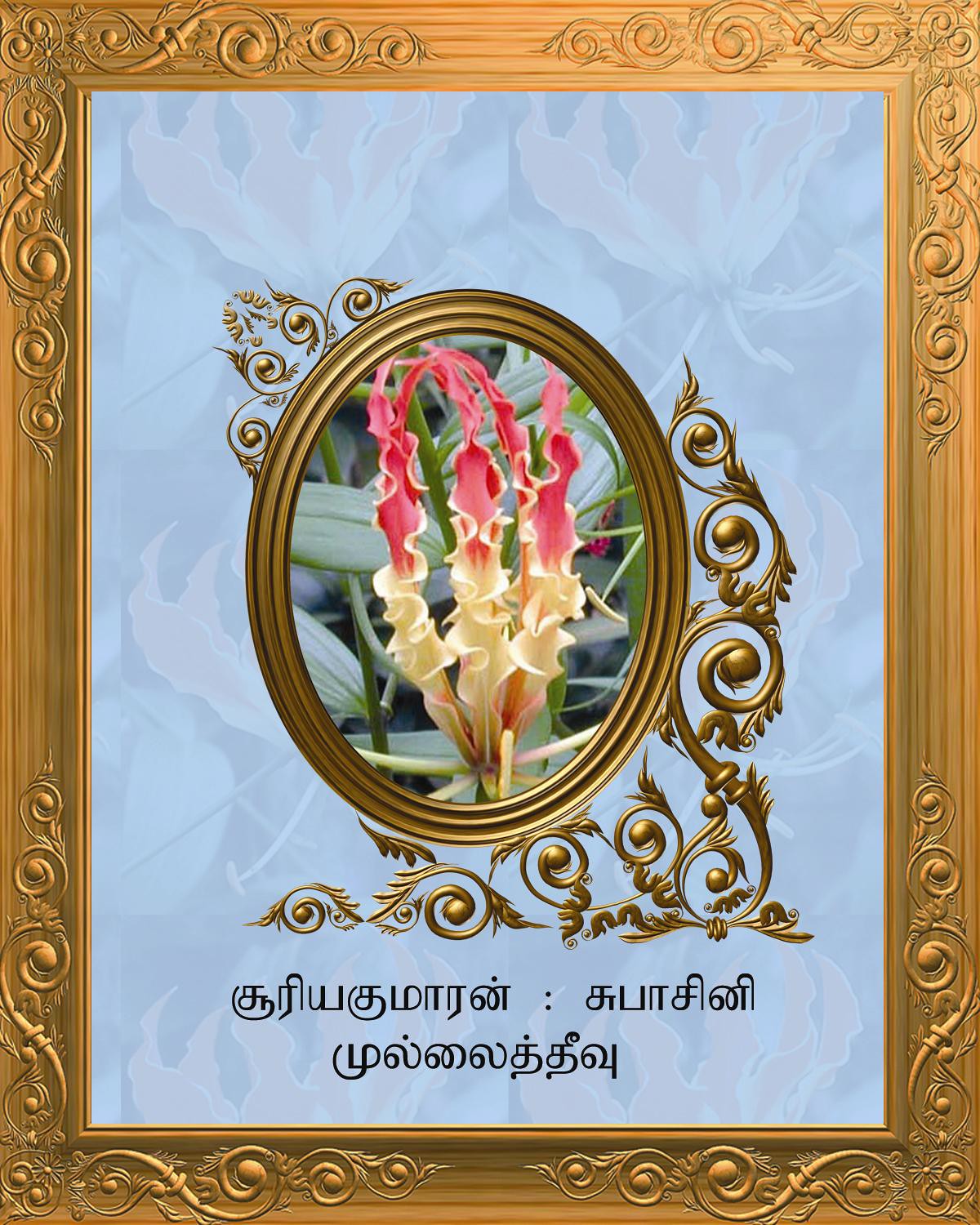This image likely depicts an ornately framed piece of art, possibly an invitation or flyer for a social event like a wedding, with text at the bottom in an Indian language. The main feature of the image is a photograph of a long, celery-like flower with red and yellow hues, set against a light blue background. Surrounding this flower is an oval-shaped, intricate golden frame that is highly ornate and designed with elaborate patterns. The flower is complemented by green leaves in the background. The entire piece is set within a larger, square, gilted gold frame that is equally elaborate in design. Additionally, the blue background of the image includes transparent flower motifs that harmonize with the gold border adorned with intricate corner designs. The overall effect is a clear, detailed, and aesthetically pleasing presentation with a mixture of blue, gold, red, and yellow tones. The framed photo appears upright, possibly meant for display on a wall, enhancing its decorative appeal.